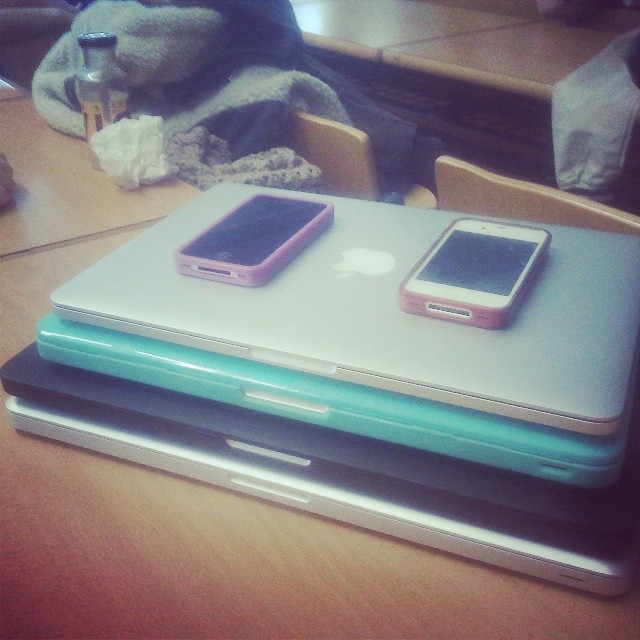The image depicts a room, likely a cafeteria or study area, featuring a stack of four different laptops on a long wooden table. Positioned prominently in the bottom right of the photograph, the laptops from bottom to top are: a silver brushed stainless laptop, a black laptop, an aqua blue or sea breeze colored laptop, and a smaller silver Apple laptop, identifiable by the visible Apple logo. On top of the stack rest two smartphones, both with pink cases, appearing to be iPhones. In the upper right quadrant of the image, another wooden table is partly visible, divided into two sections with a piece of cloth hanging off its bottom right corner. To the upper left, there is a chair draped with a pile of coats or jackets, partly obscuring it. Nearby, on another set of wooden tables, sits a glass bottle with a crumpled white napkin beside it. The setting is enriched with various details hinting at a study or work environment, potentially occupied by students, given the scattered personal items like jackets and the presence of technological gadgets.